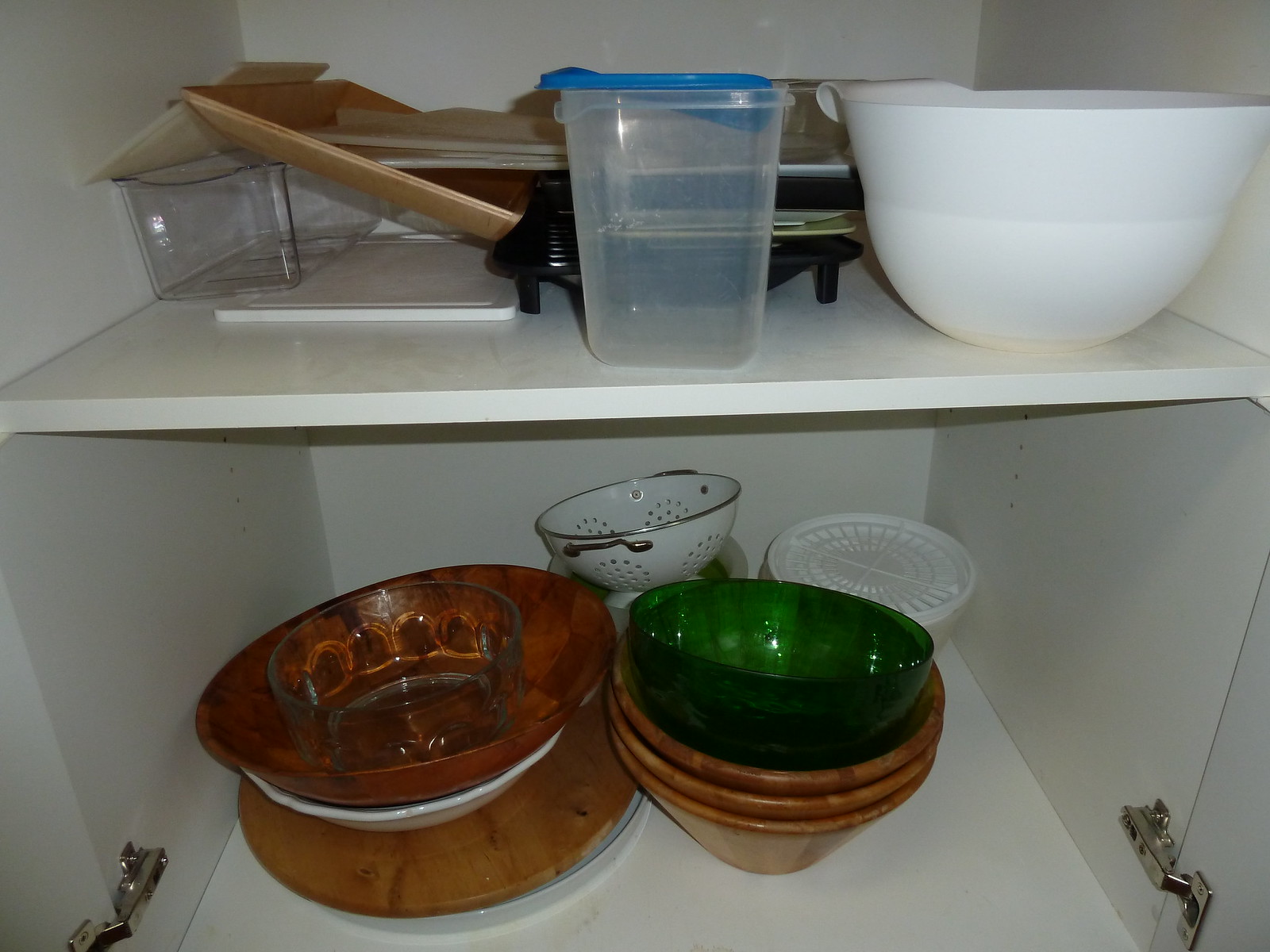This photograph captures the interior of a kitchen cupboard with pristine white walls and a matching back panel, flanked by partial views of two silver hinges on either side. The cupboard houses two shelves laden with various kitchen items. 

The top shelf is a picturesque assembly of culinary paraphernalia, featuring two white plastic bowls nestled among an assortment of objects. A clear, tall plastic container with a distinctive blue lid stands prominently towards the front, partially obscuring a piece of tile resting behind it. Scattered around are some pieces of paper, another clear plastic container missing its lid, and a mysterious black item, partially concealed by the tall container.

On the bottom shelf, four bowls—three brown and one green—are arranged in a neat cluster. To their left, a wooden platter rests beside a white tray, atop which a multicolored brown bowl is stacked on a white bowl. Towards the rear of this shelf, a white metal colander and a white plastic strainer complete the orderly yet diverse array of kitchenware.